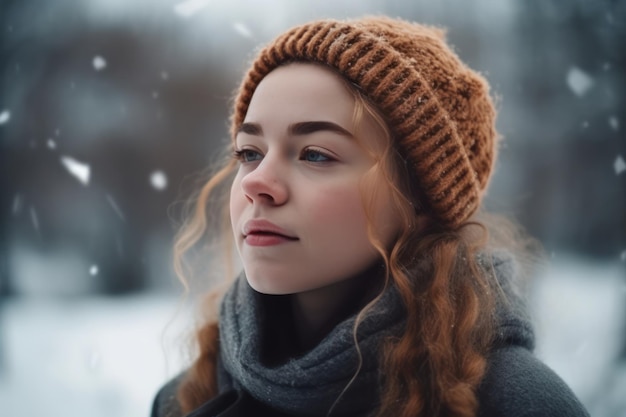In the image, a striking woman stands amidst sporadically falling snow, with a blurred background that hints at shadowy buildings, making it impossible to discern whether it's a small town or a city. The woman has reddish-brown, wavy hair that frames her fair face and falls over both shoulders. She wears a thick, brown knit hat, rolled up at the edges, perfectly matching the hue of her hair and partially revealing her forehead. Her blue eyes, accentuated with eye shadow, gaze into the distance with a sad, half-smile and her lips slightly parted. Her cheeks and nose are rosily flushed, complementing her heavily made-up look, yet her overall appearance remains natural. She is dressed warmly in a gray scarf and a dark gray jacket, fitting for the wintry day.